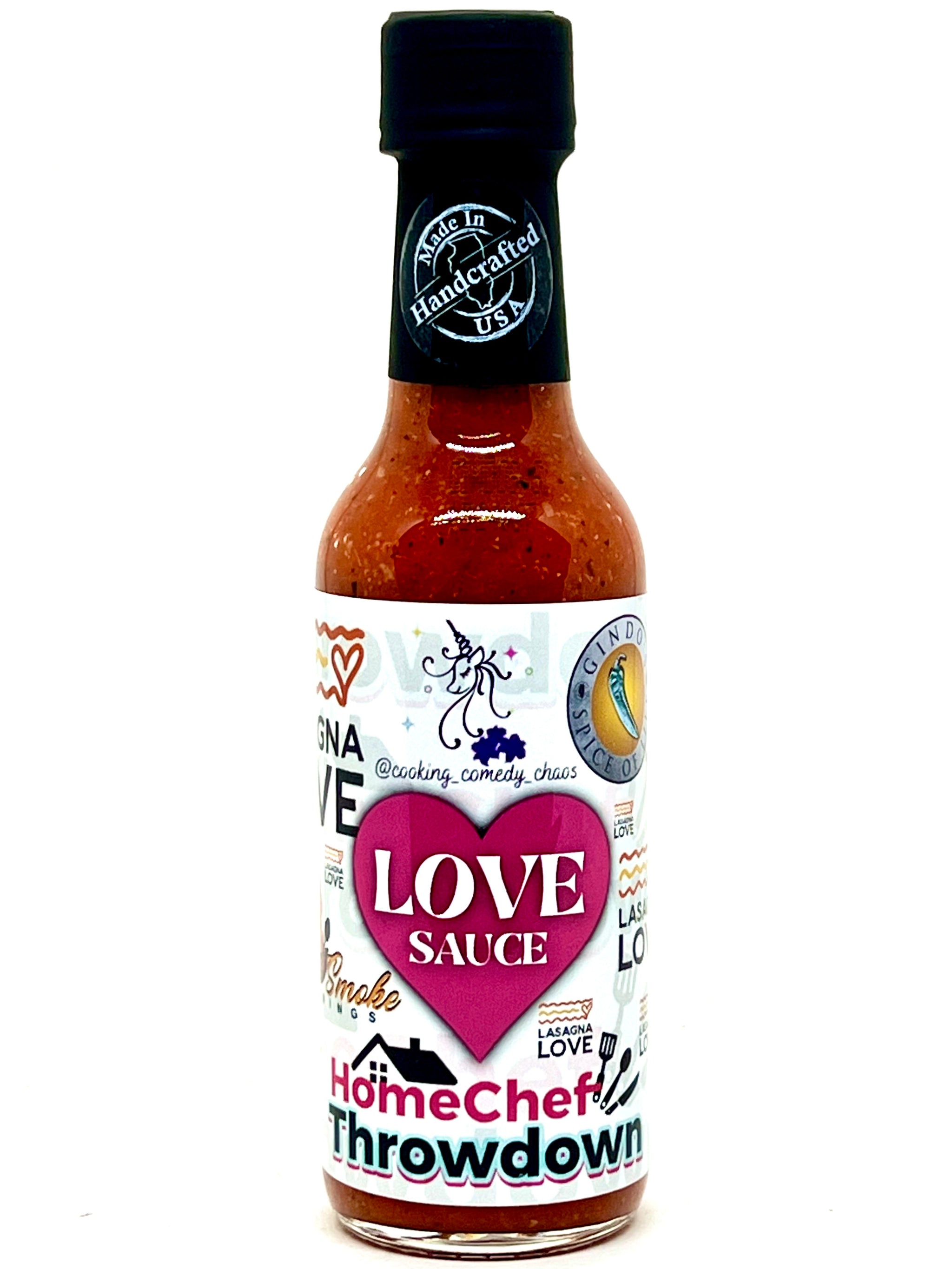The image features a tall, narrow bottle of sauce with a tapered neck and a black sealed cap. The transparent bottle reveals an orange, grainy sauce with small black and white flecks. Just below the cap is a black label displaying a circular white stamp that reads "Made in USA" around the border, with "Handcrafted" in the center. The bottle's main label is predominantly white, featuring a central reddish-pink heart shape with the words "Love Sauce" inside. Below the heart, there is a graphical representation of a house roof next to the text "Home Chef" printed in pink, and "Throwdown" in black. The bottle appears to float against a clear, white background, emphasizing its shape and details in a style that blends Photographic Representationalism and Realism.